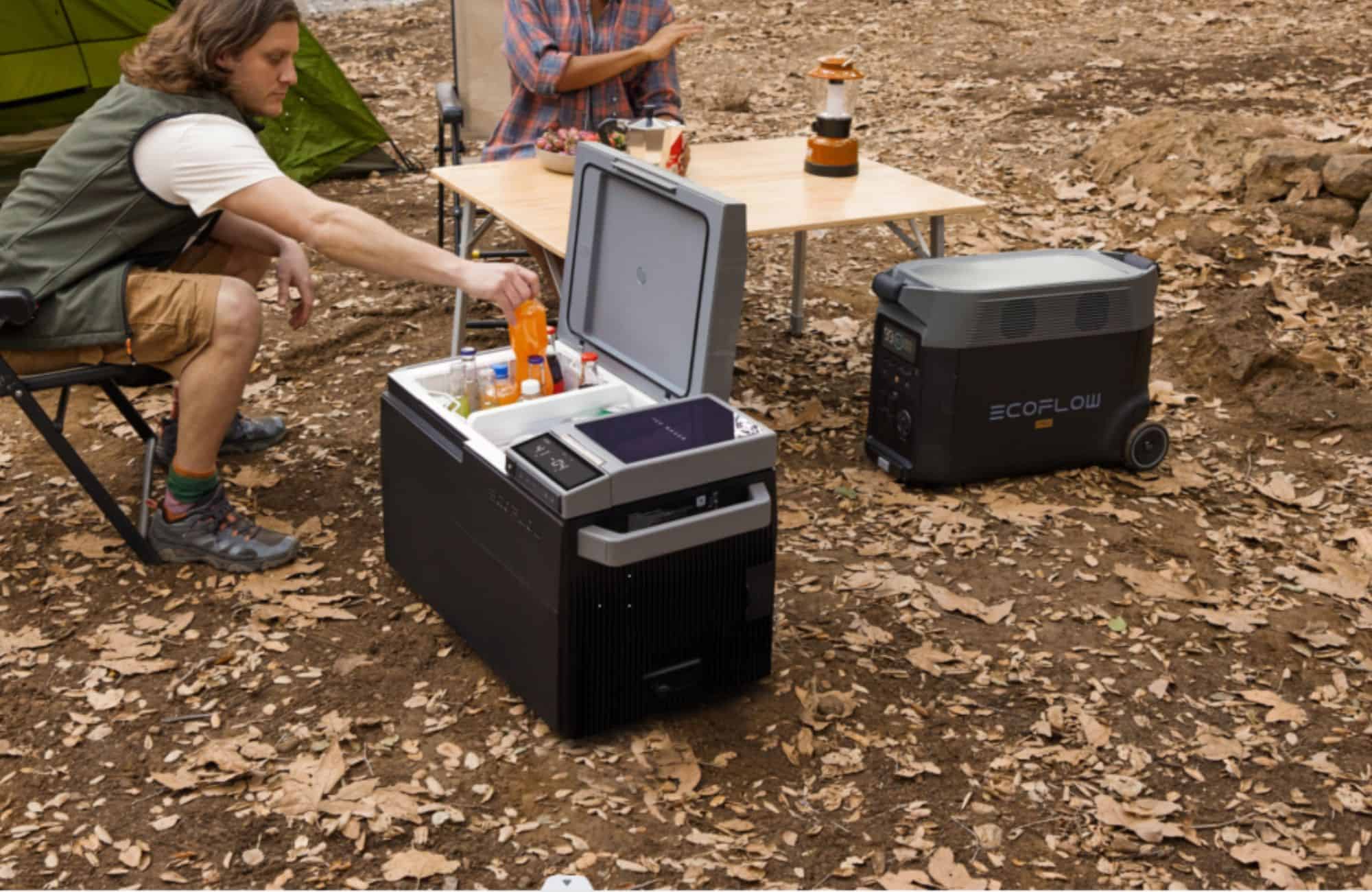The image captures a candid outdoor camping scene, likely set during the fall in a forested area with dried leaves scattered on a muddy forest floor. A man with shoulder-length, wavy light brown hair, is seated in a folding chair on the left side of the photo. He wears a white t-shirt under a hunter green vest, knee-length brown cargo shorts, and gray athletic shoes with green and pink socks featuring an orange band. He is reaching into a large, modern black cooler with a white interior, extracting a bottle of orange soda. Adjacent to this cooler, there is another high-tech cooler labeled "EcoFlow," which has handles and wheels.

Further to the right, a woman, with her head out of the frame, is sitting at a foldable camp table. She wears a blue and pink plaid shirt with rolled-up sleeves, exposing her tan arms, and is seated in a tan chair. The table holds a camping lantern, a moka pot, and a bowl of food, indicating that a meal is in progress. In the background, a green tent and some gray rocks can be seen, contributing to the wilderness environment. The lighting is diffuse, suggesting an overcast day with scattered, subdued light.